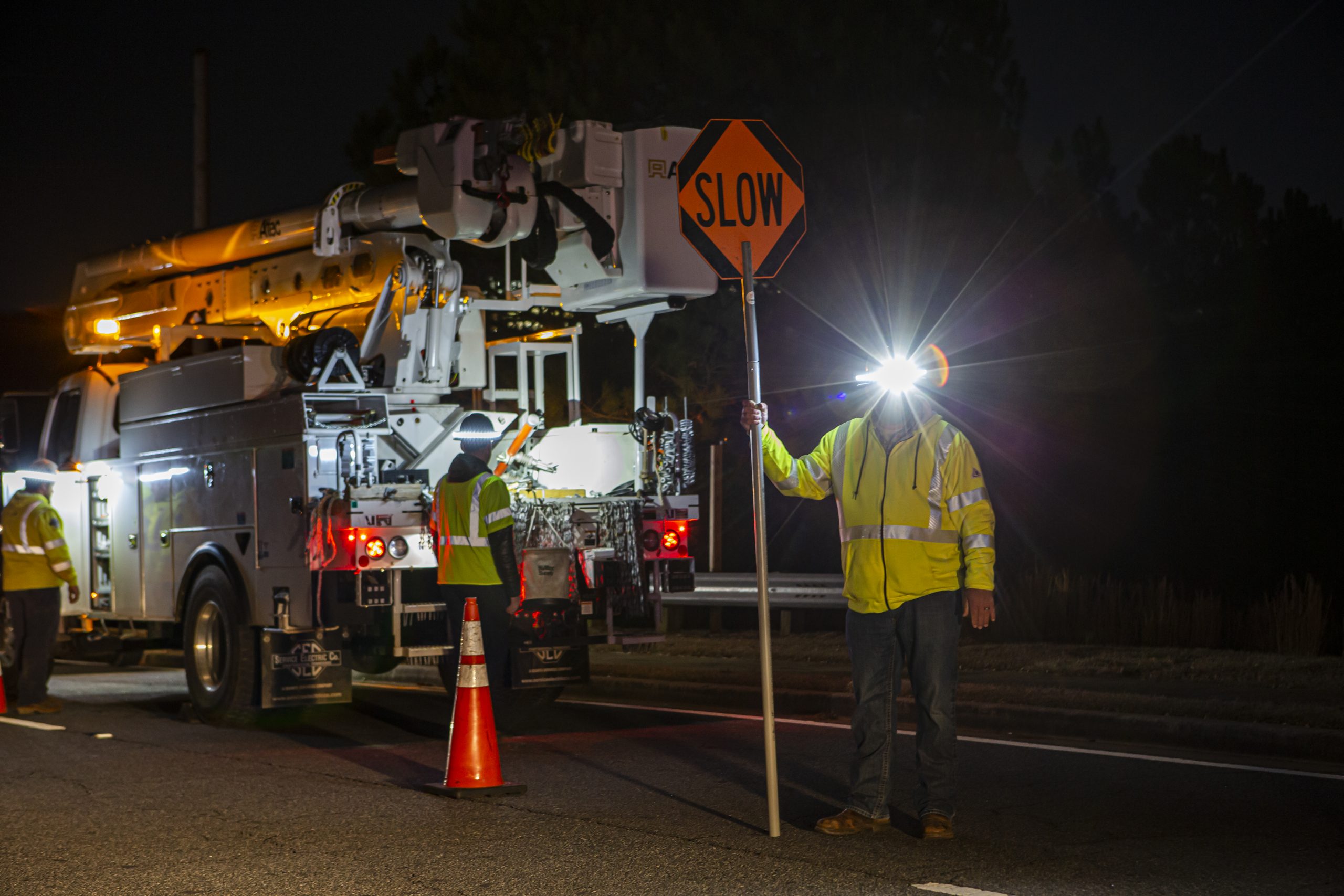This nighttime color photograph captures a road work scene featuring a large utility truck and three men clad in yellow reflective safety jackets with metallic stripes. The man to the right stands under an intense, star-bursting light that obscures his face, while he holds an orange "SLOW" sign on a long pole to direct traffic. He is dressed in a long-sleeve protective jacket and denim jeans. To his left, another worker stands at the back of the truck by an orange safety cone with two white stripes. This man is also in a yellow reflective jacket and appears to be retrieving something from the truck's open doors. The utility truck itself has glowing taillights and is equipped with an elevated basket for reaching high places, presumably for electrical work. Further left, the third worker, similarly dressed, stands near the truck. The dark night sky serves as a backdrop, highlighting the illuminated scene on the road.